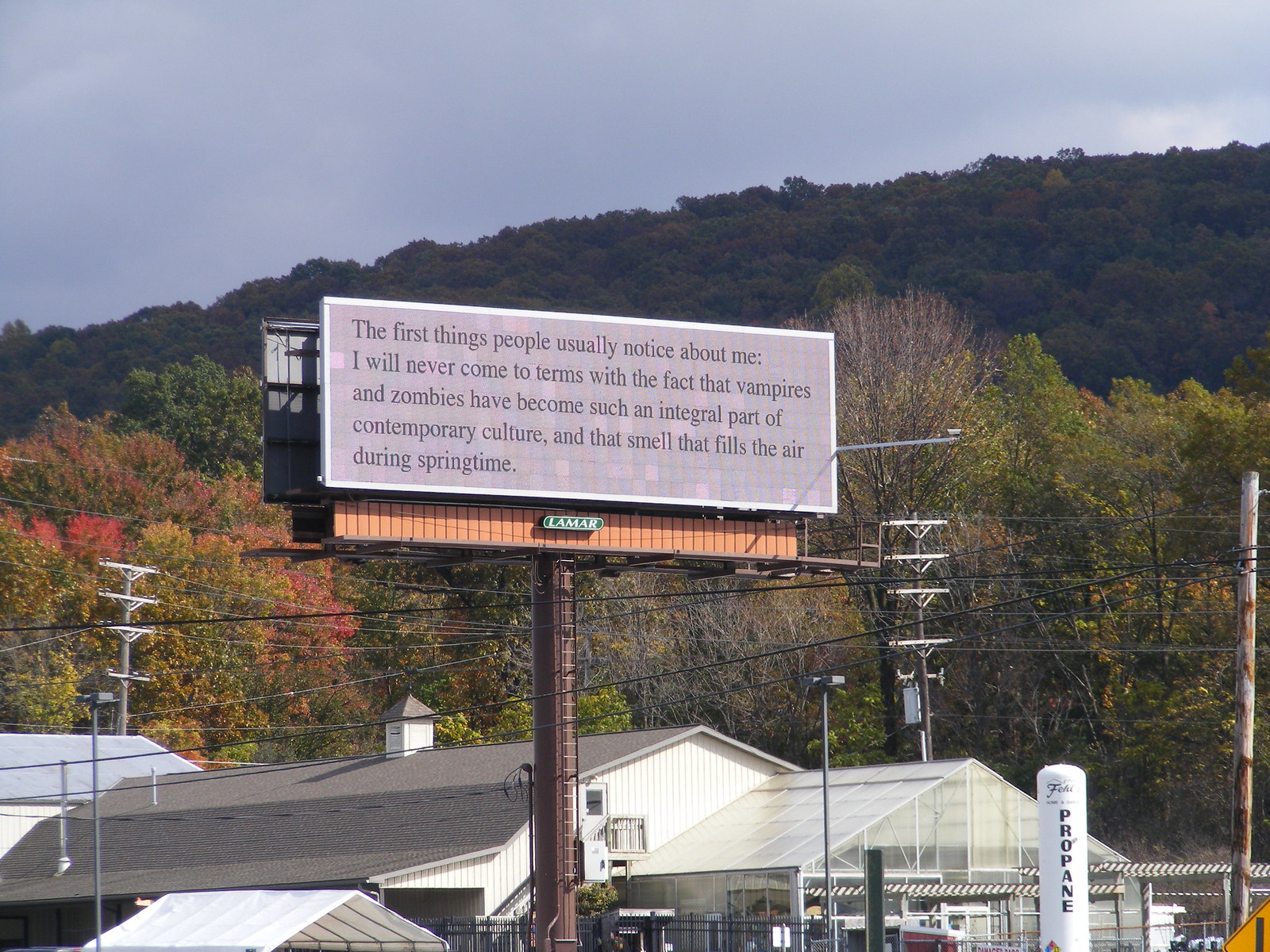In the foreground of the image, a colossal billboard dominates the scene. This advertisement board, prominently placed beside a large metal post, features an intriguing text on a vivid purple background. The quirky message reads, "The first things people usually notice about me. I will never come to terms with the fact that vampires and zombies have become such an integral part of the contemporary culture, and that smell that fills the air during springtime." Below this, the billboard has a smaller orange sign with the name "Lamar" on it.

The backdrop of the image offers a serene, outdoor setting. In the distance, there is a rolling hill beneath a grayish-blue sky. A variety of trees create a rich tapestry—some boasting lush green foliage, while others display vibrant red and yellow leaves or stand bare. Beneath the tree line, an array of electrical wires spans the scene, supported by visible poles and crossbars.

At the foot of the hill lies a large white building featuring a greenhouse attached to the right side. Adjacent to the greenhouse is an impressively tall propane tank, nearly matching the building's height. To the left, a structure with a barn-shaped roof stands out, its white exterior contrasting with its black roof. All these elements come together to create a picturesque setting for the attention-grabbing billboard in the foreground.